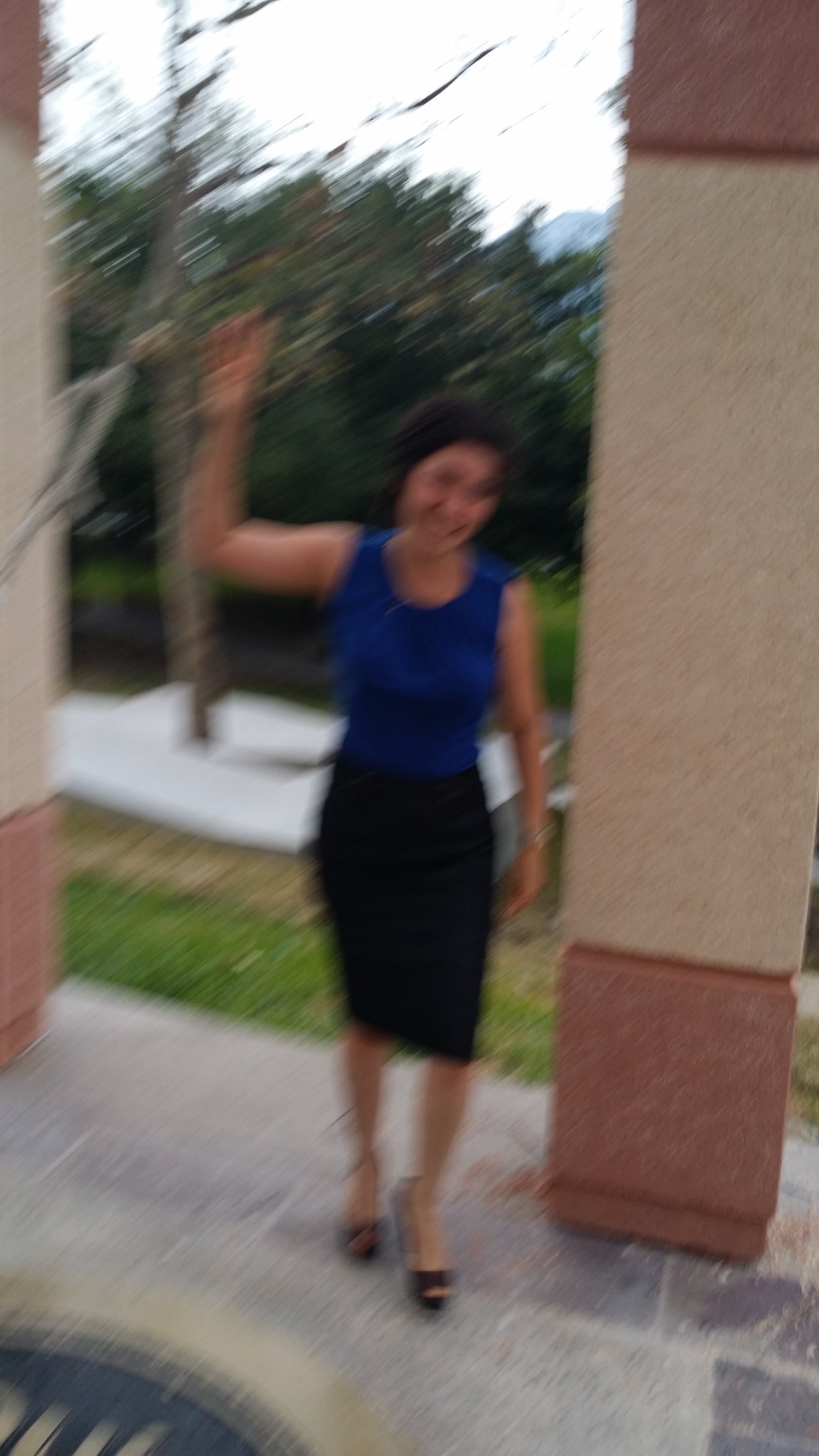In this very blurry image, a woman with a fair to medium complexion and short dark hair is depicted standing with her right arm raised at a perfect right angle, as if waving awkwardly. She is wearing a sleeveless dark blue blouse paired with a black pencil skirt and black high heels. Her left arm, adorned with what looks like a silver watch, hangs by her side.

The setting appears to be a porch or entryway with distinctive paving made up of brick-like or slate tiles. She is between two tall, two-tone columns or pillars. These columns are constructed with a reddish-brown base and top, and the middle section is tan or beige, extending taller than the woman herself. The ground features a circular emblem, consisting of a black oval with a gold border and possibly gold writing, suggestive of a hotel logo or similar design.

In the background, tall trees and some form of white tarp or cloth are visible, indicating an outdoor area. The sky is overcast, and there might be a glimpse of a mountain range in the distant corner. Despite the blurriness, the woman seems to be smiling lightly, adding to the vibrant yet mysterious aura of the scene.